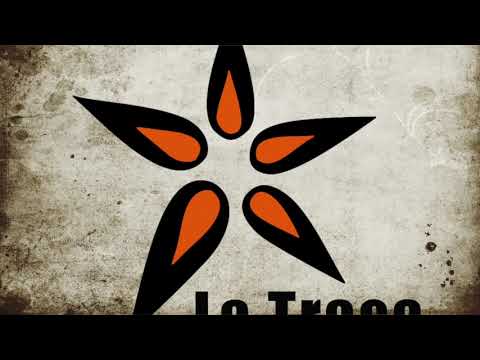The image appears to be a screenshot from a video, specifically a horizontally aligned rectangular frame flanked by thick black borders at the top and bottom. The main focus is a logo-like design partially obscured by the bottom border, showing fragmented letters that could spell "Le Tro" or "L-O T-R," though the exact text remains unclear. Central to the image are five teardrop shapes, reminiscent of flower petals or a five-pointed star, intersecting at their rounded ends. These shapes are primarily black with smaller vibrant orange teardrops nested within each. The backdrop is a textured, weathered gray surface with patches of black and brown, resembling a dingy, aged cement wall typical of outdoor concrete structures. The overall image gives an impression of being mid-transition, either zooming in or out, emphasizing the dynamic and fragmented nature of the scene.